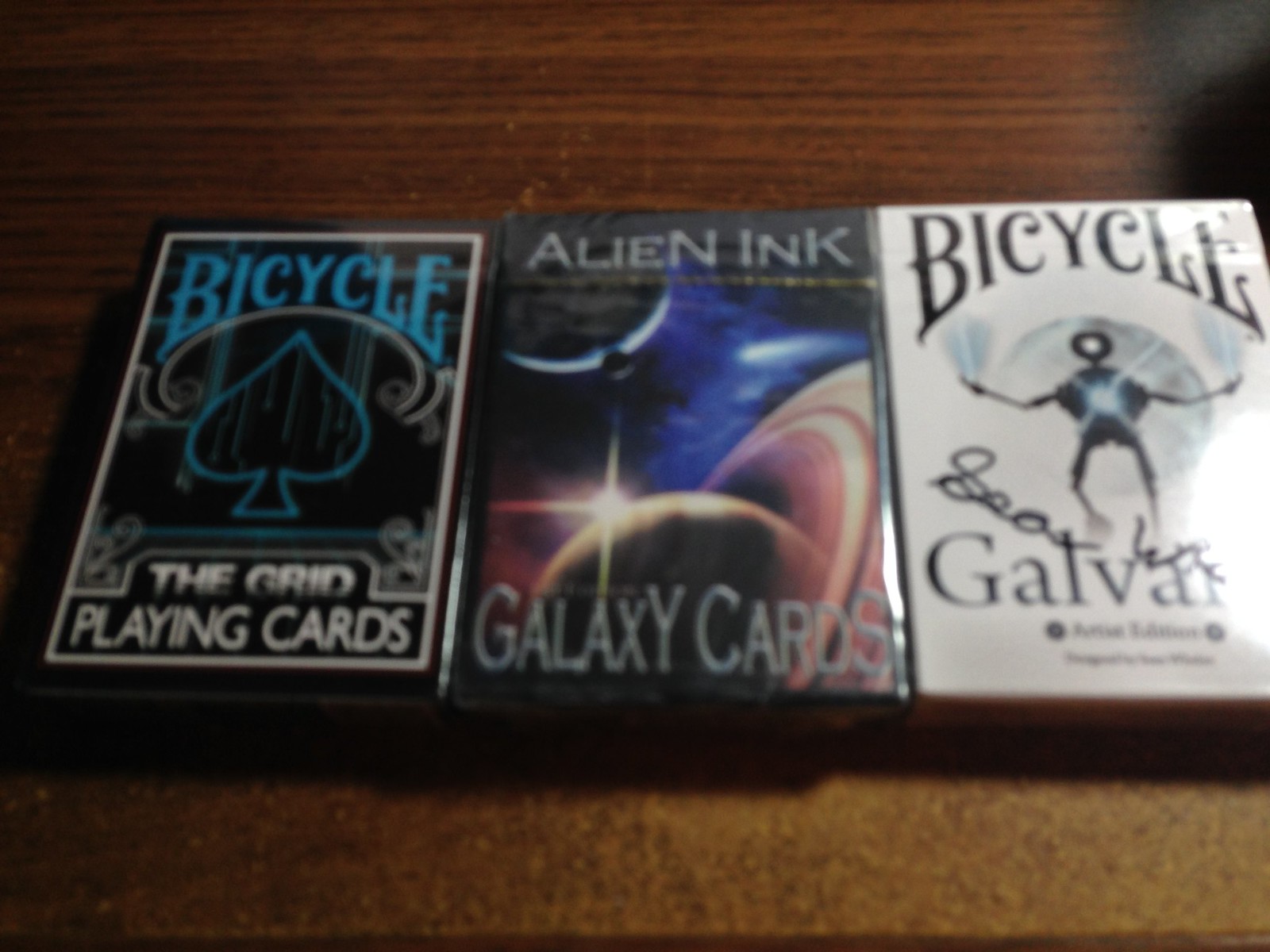The image depicts three distinct packs of playing cards, each unopened, arranged on a dark brown table. The table's surface varies in condition; the upper portion appears smooth, displaying the wood grain in rich, dark brown or black hues, whereas the lower section is coarser, seemingly sanded down to bare wood, revealing a distorted, less smooth texture.

Centrally positioned are the three decks of cards. The leftmost deck is black with blue text that reads "Bicycle," featuring a blue spade symbol and labeled "The Grid Playing Cards." The middle deck is another black box titled "Alien Ink Galaxy Cards" in white or silver lettering, adorned with a galaxy image at its center. The rightmost deck is housed in a white box with "Bicycle" inscribed in black. It showcases an illustration of a robot with a blue beam emanating from its chest. The term "Galva" is partially visible, and the box appears to be signed in black marker, though the signature's details are unclear.